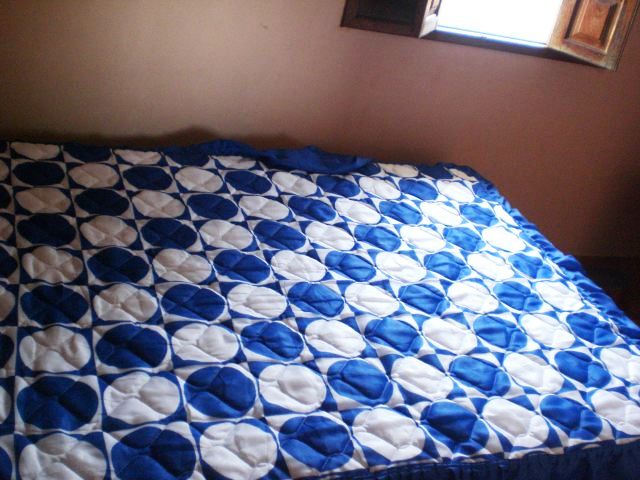The photo depicts a small bedroom corner with a bed positioned against a light tan or beige wall. The bed has a blue and white bedspread featuring a grid-like checkerboard pattern made up of alternating blue and white squares. Each square contains a contrasting colored circle—white circles within blue squares and blue circles within white squares. The bed, which appears to be either a queen-sized mattress lying directly on the floor or a low bed frame, is illuminated by natural sunlight streaming through an open window located in the upper right portion of the photo. The window has wooden blinds pulled to the sides, allowing bright white light to fill the room and cast a natural glow over the end of the bed. The image is taken at an angle, focusing downwards towards the bed, giving a partial but clear view of the scene.